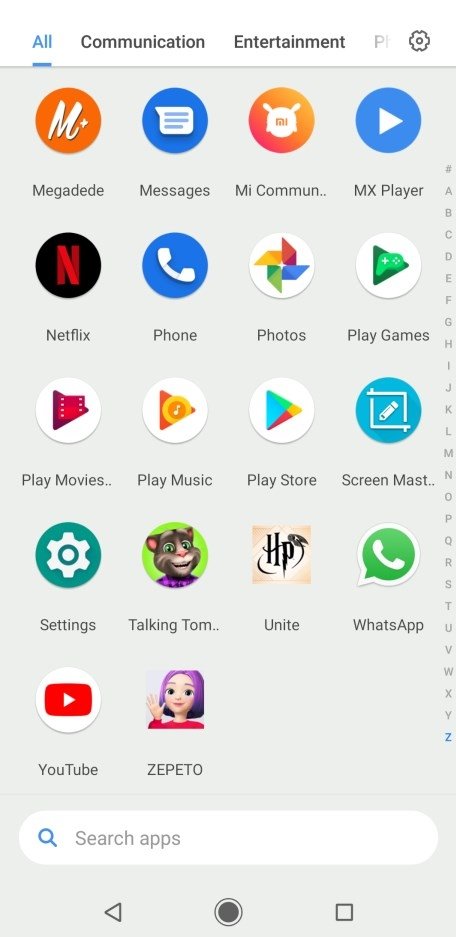The image showcases a digital interface with various application icons arranged in a grid. 

At the top of the interface, there are several tabs: "All," "Communication," "Entertainment," and a settings icon on the extreme right. The "All" tab is highlighted in blue while the others are written in black.

The applications are represented with distinct icons:
- **Megadeth**: Orange icon.
- **Messages**: Blue icon with a white conversation box.
- **Mi Communication**: Orange icon with "MI" in the center.
- **MX Player**: Blue icon with a white play button.
- **Netflix**: Black icon with a red "N".
- **Phone**: Blue icon with a white phone symbol.
- **Photos**: White icon with a multi-colored propeller (red, yellow, green, and blue).
- **Play Games**: White icon with a green play button and joystick.
- **Play Movies**: Icon with a purple play button and movie symbol.
- **Play Music**: Icon with an orange and yellow play button alongside a music note.
- **Play Store**: White icon with the play logo in multiple colors.
- **Screen Master**: Light blue icon with a square and a pen.
- **Settings**: Green icon with a white gear.
- **Talking Tom**: Green icon with a cat figure.
- **Unite**: Brown icon with "HP".
- **WhatsApp**: Green icon with a white speech bubble and phone.
- **YouTube**: Red icon with a white play button.
- **A Pet**: An icon with a character having purple hair, waving, and wearing a red T-shirt.

At the bottom of the screen, there is a search bar labeled "Search apps" accompanied by a blue search button on the bottom left. The background of the interface is white, providing a clean and organized layout for easy navigation.